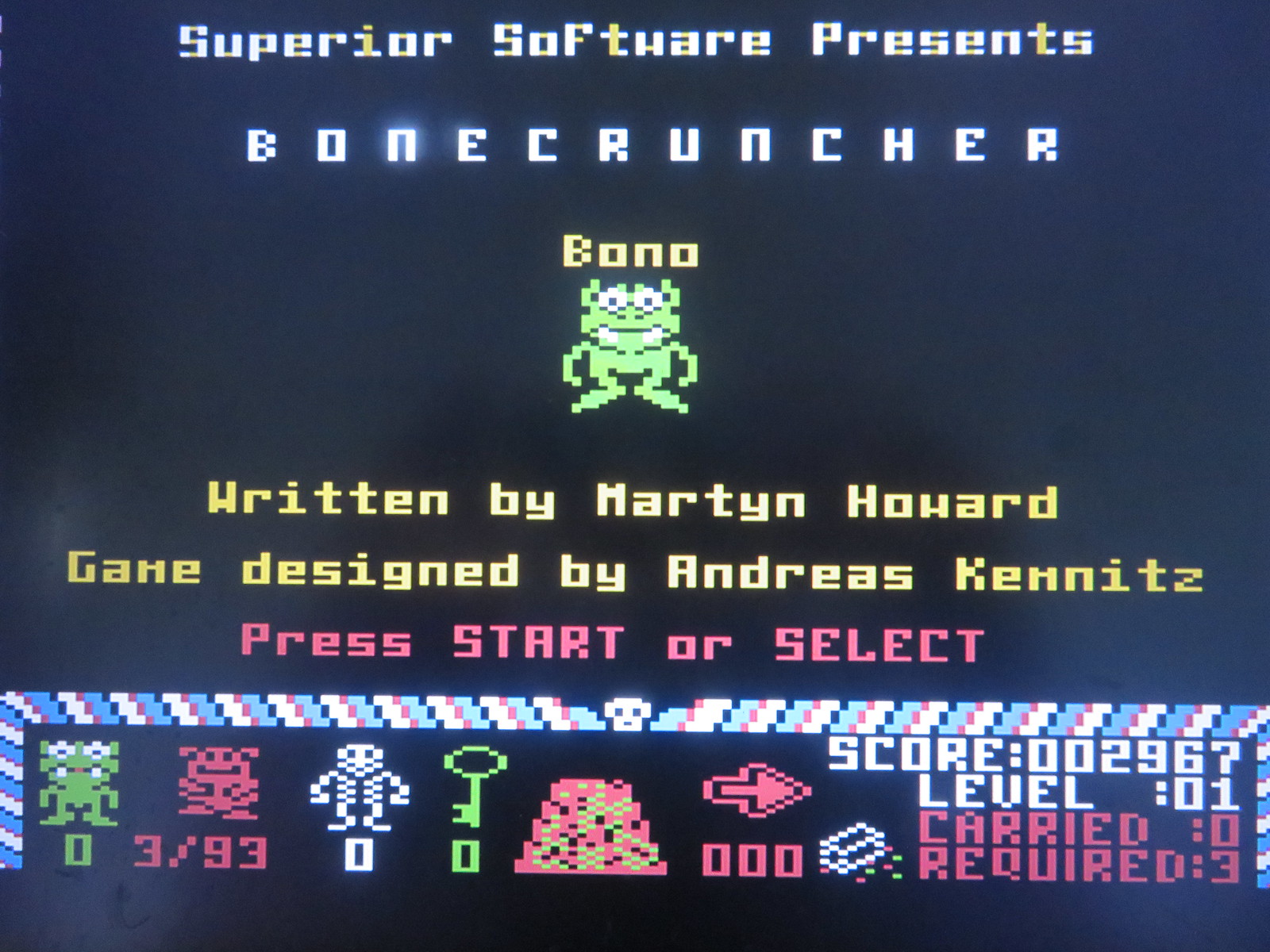The image is a detailed screenshot of a vintage video game start screen for the game "Bone Cruncher" by Superior Software. The background features a dark navy blue gradient, fading to a lighter shade towards the lower left and right corners. At the top, in an old video game font with striped white and yellow, it says "Superior Software Presents." Below that, in all caps and glowing white letters, it reads "BONE CRUNCHER." Underneath, in yellow letters, the character name "Bono" is prominently displayed. 

Central to the image is a green, pixelated cartoon character that resembles a frog-like monster, highlighting the early digital art style. Further down, yellow text indicates that the game was written by Martin Howard and designed by Andreas Kennitz. In pink letters, the instructions "Press Start or Select" invite interaction.

Towards the bottom, there's a multicolored scoreboard displaying different figures, a key, and various icons. The numbers "0, 3/93, 0, 0" are shown, along with a pyramid-like shape, a right arrow, and the score "002967." Additionally, details such as "Level 01," "Carried: 0," and "Required: 3" are included. The imagery and text exhibit a distinctive 8-bit style, with noticeable pixels that enhance its vintage aesthetic.